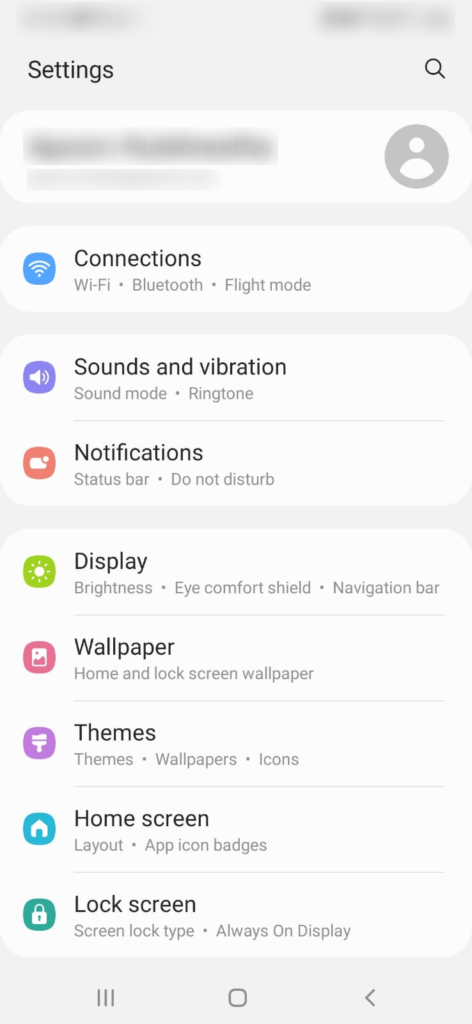The image displays the settings section of an Android phone. At the top, personal information is blurred out, leaving only the "Settings" label visible alongside a person icon on the right. Adjacent to "Settings," there is a magnifying glass on the right side of the screen. The background is a light yellow, complemented by white fields that contain important information.

In the "Connections" section, there are options for Wi-Fi, Bluetooth, and Light Mode, indicated by white icons against a blue background, including a signal icon. The "Sound and Vibration" section follows, containing settings like Sound Mode and Ringtone, represented by a speaker icon on a purple background. The "Notification Status Bar" features a Do Not Disturb option with an indistinct orange icon.

Next is the "Display" section, which offers settings for Brightness, Eye Comfort Shield, and Navigation Bar, marked by a green icon with a white sun. The "Wallpaper" section highlights options for the Home and Lock screen wallpapers, displaying an image of mountains and the sun on a pink background.

The "Themes" section, including Wallpapers and Icons, is depicted by a vertical paintbrush on a purple background. The "Home Screen" section allows adjustments to layout and app icon badges, symbolized by a small home on a blue background.

Below this, the "Lock Screen" section shows options for Screen Lock Type and Always On display, represented by a lock icon on a green background. At the bottom of the phone screen are the three standard navigation buttons: Close, Back, and Home.